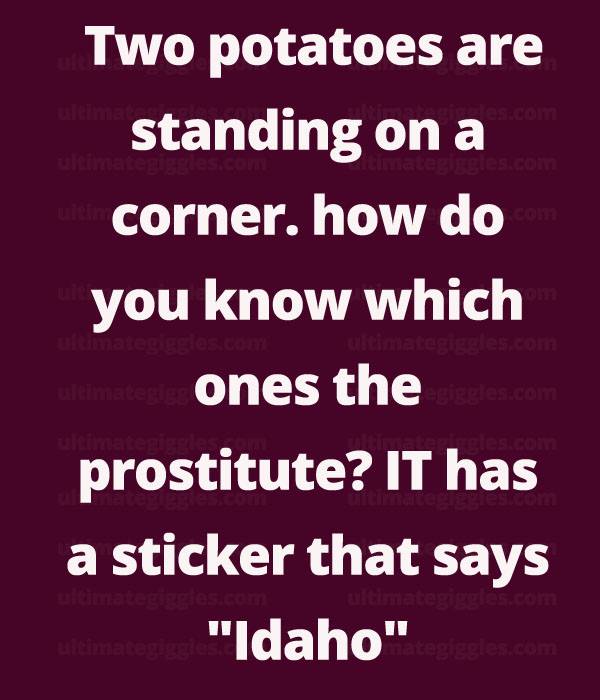The image features a solid background in a deep, plum aubergine color with a repeated, light watermark that reads "ultimategiggles.com." Superimposed on the background in bold, white sans-serif font is the text:

"Two potatoes are standing on a corner. How do you know which one is the prostitute? It has a sticker that says Idaho."

The phrase is a joke, playing on the pun between "Idaho" and "I da ho." The overall design suggests it’s a meme graphic commonly shared on social media platforms like Facebook. The text appears to have been hastily typed, evident from the lowercase "h" in "how."